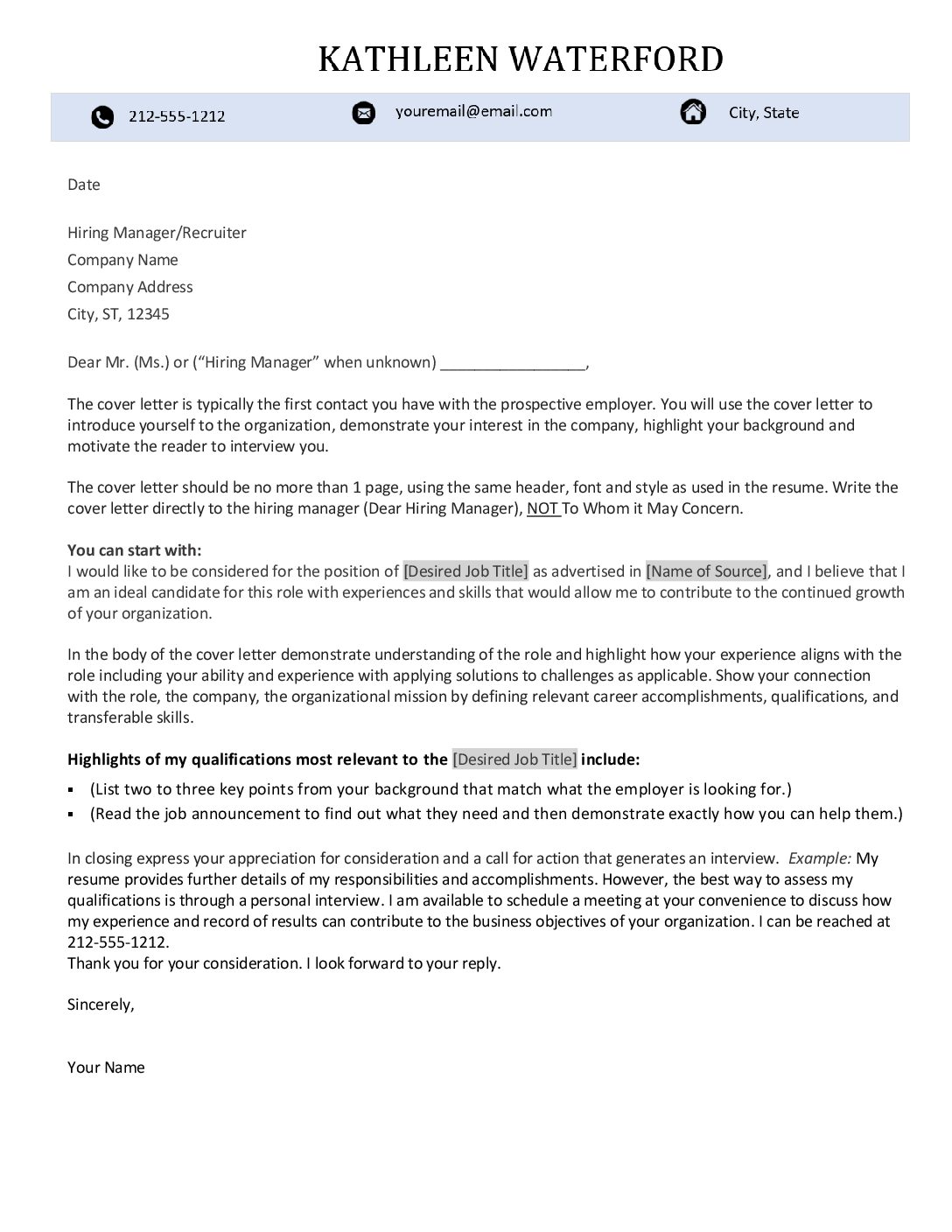The image contains a detailed example of a professional letter template on a clean, white background. At the top, "Kathleen Waterford" is prominently displayed in bold black letters. Below this, a gray box features an organized layout: a phone symbol followed by a phone number, an envelope icon accompanied by an email address at the center, and a home icon with a specified city and state to the right.

In the top left section, just beneath the gray bar, the template begins with a formal structure: it starts with "Date" followed by "Hiring Manager / Recruiter." Next are placeholders for "Company Name" and "Company Address," ending with "City, State 12345." The salutation reads: "Dear Mr. or Mrs. [or Hiring Manager when unknown]," followed by some blank space designated for the main body of the letter.

The letter proceeds with a brief introduction stating, "This is typically the first contact you have with the prospective employer." Further down, a section marked as a guide suggests ways to begin the letter with "You can start with..." and offers relevant titling advice. The letter then includes a portion for highlighting qualifications relevant to the desired job title, concluding with instructions on how to properly close out the letter. The template appears to be a comprehensive guide for crafting a professional job application letter.